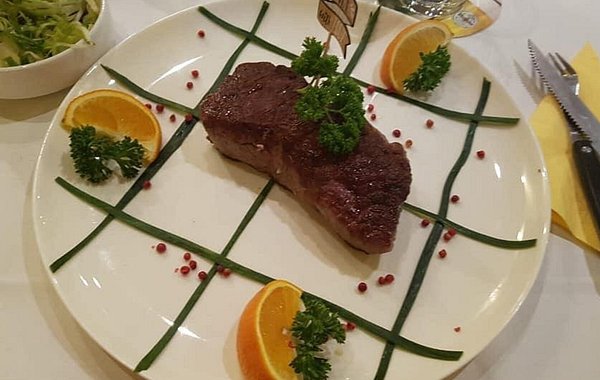This close-up, Instagram-style image captures a beautifully arranged dish on a pristine white ceramic plate, set against a white table. At the plate's center lies a well-done piece of steak, crowned with a tuft of fresh parsley and a decorative toothpick. Surrounding the steak, three orange wedges form a triangle, each accompanied by a sprig of parsley. The plate is artistically adorned with long green strands, possibly cucumber, laid out in a tic-tac-toe pattern. Scattered across this layout are small red balls or seeds, adding a splash of color. To the right of the plate, a yellow napkin is neatly placed with a fork and knife aligned in classic dining style. To the left, a round white ceramic bowl holds a fresh salad of assorted greens, completing the sophisticated dining setup.